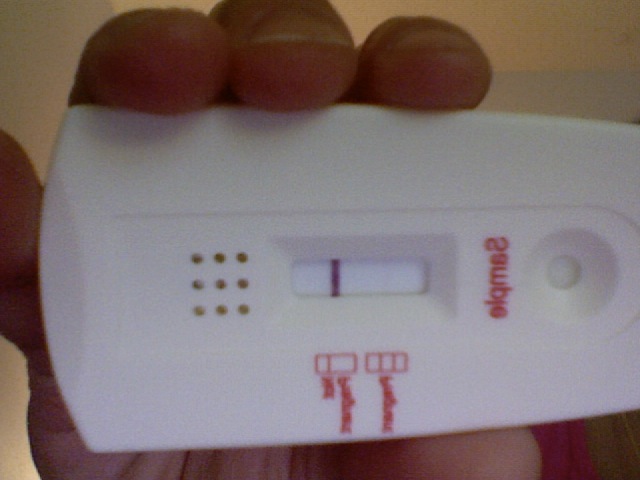In an indoor setting, this detailed photograph captures a white, hard plastic test device, potentially either a pregnancy or COVID test. The product name, starting with the letter "S," is displayed in reversed red letters. The test device features nine small holes in the center and a window indicating test results. Inside the window, a piece of fabric displays a single, straight purple line, implying a specific result. The device's circular top continues the fabric piece. The test is held delicately by the first three fingers, with the pinky resting at the back bottom and the thumb positioned below the device. A diagram on the device distinguishes between a single line and a double line for result interpretation; currently, only one line is visible.